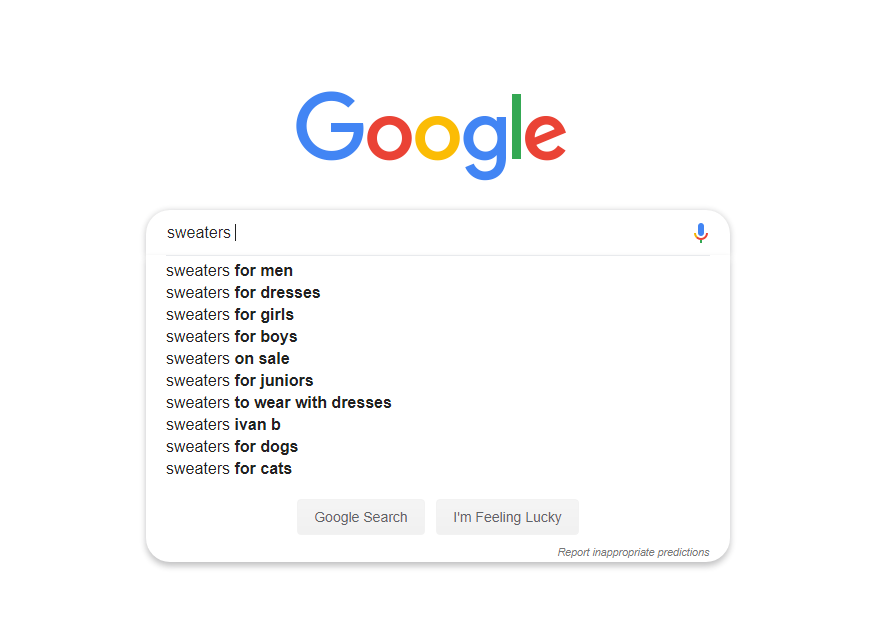This is a screenshot of the Google search homepage captured in landscape orientation, blending seamlessly with the surrounding web page. The image is characterized by its typical dimensions, being wider than it is tall. At the top of the image, the iconic Google logo is displayed, featuring a blue capital "G", a red "o", a yellow "o", a blue lowercase "g", a green "l", and a red "e" - all in their standard colors and order.

Below the logo sits the familiar search bar, in which the user has typed "sweaters". Positioned to the right of the search bar is the blue microphone icon, indicating the option to use voice search. A drop-down menu is visible beneath the search bar, showcasing possible search suggestions. These suggestions include:
- sweaters for men
- sweaters for dresses
- sweaters for girls
- sweaters for boys
- sweaters on sale
- sweaters for juniors
- sweaters to wear with dresses
- sweaters Ivan B
- sweaters for dogs
- sweaters for cats

At the bottom of the screenshot, two rectangular gray buttons are visible - the left one labeled "Google Search" and the right one labeled "I'm Feeling Lucky".